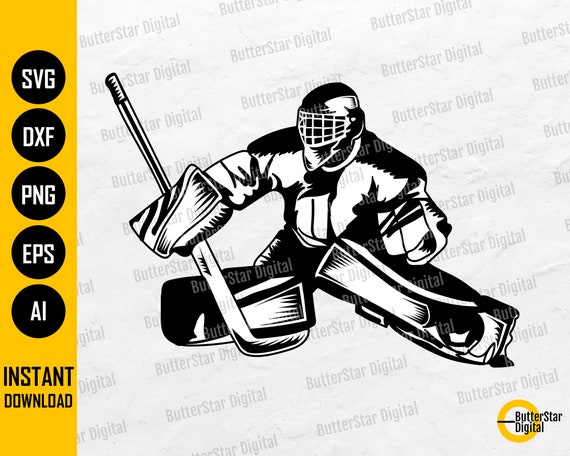The image is a black and white sketch of a hockey player, likely a goalie due to the extra knee pads and face cover. The goalie is looking to the left with his knees pointing towards each other, suggesting a defensive stance to block a puck, which is not visible in the image. The entire image is watermarked repeatedly with the words "Butterstar Digital," which also appears prominently across the goalie in a faded gray color. In the bottom right corner, a dark black area contains a yellow circle. On the left edge, a yellow bar runs downwards, and below it, in all capital letters, it reads "INSTANT DOWNLOAD." Above this text, five equally-sized black circles, stacked vertically, display the file formats "SVG," "DXF," "PNG," "EPS," and "AI" in white capital letters. The goalie's face is entirely covered by his helmet, obscuring any facial expression.